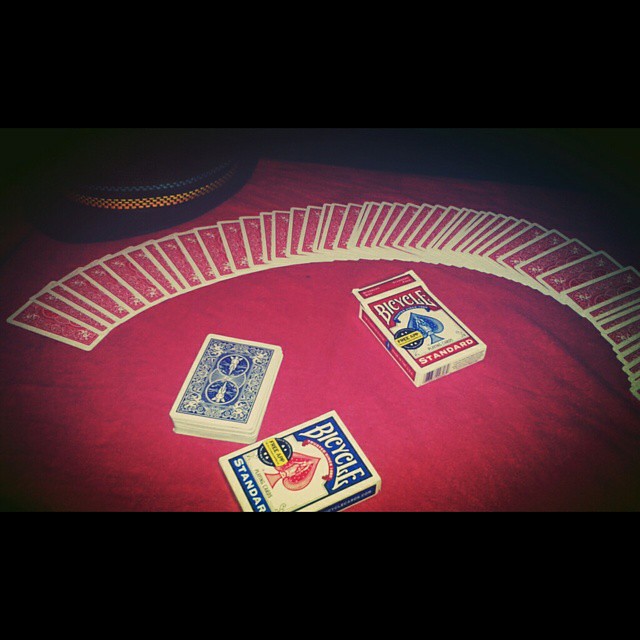This image showcases a meticulously arranged display of playing cards on a vibrant red playing table. The background at both the top and bottom of the image is a stark black, creating a dramatic contrast. At the bottom center of the image is a sealed blue deck of Bicycle brand playing cards. The deck's packaging features "Bicycle" in prominent white text, a red spade logo in the center, which is encased in a dark blue emblem marked by a yellow stripe, and the word "Standard" at the bottom.

Above this blue deck lies a fully visible deck of cards positioned face down, displaying an intricate dark blue back design. The design comprises two circular motifs surrounded by elegant white linework. To the right, we see another package of Bicycle playing cards, but this one is red and open. The red deck retains the same "Bicycle" branding and "Standard" text, but features a blue spade logo instead. The red cards are dramatically fanned out, spanning almost the entire width of the table, showcasing their intricately lined backs. To the top left corner of the image, there's a black fedora with a stylish gold stripe adorning it, adding an intriguing element to the composition.